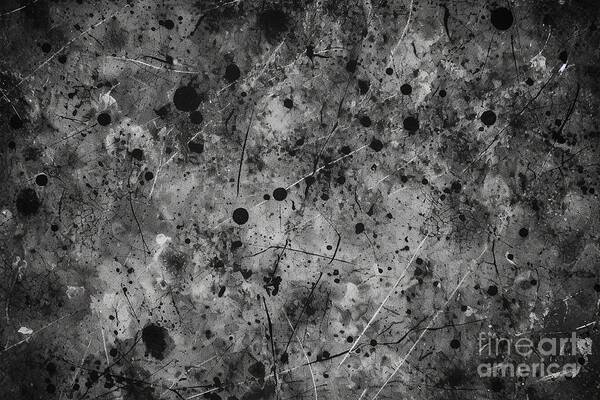This image is a detailed close-up of abstract fine art, presented by Fine Art America, as noted in muted gray text at the bottom right-hand corner. The artwork features a spectrum of muted tones, predominantly shades of gray and black, with occasional highlights of white. The canvas appears as if various colors of paint were splattered and flung across a black background, creating an intricate pattern of black, gray, and white dots intermingled. The predominant color is gray, reminiscent of smoke weaving through the image, with black dominating the corners. Thin, scattered black and gray lines add texture, giving the impression of striations and markings like those found on bundled and flattened paper. The overall composition is abstract, with no discernible objects or figures, characterized by ink blot-like black spots and a mottled interplay of gray and black hues.